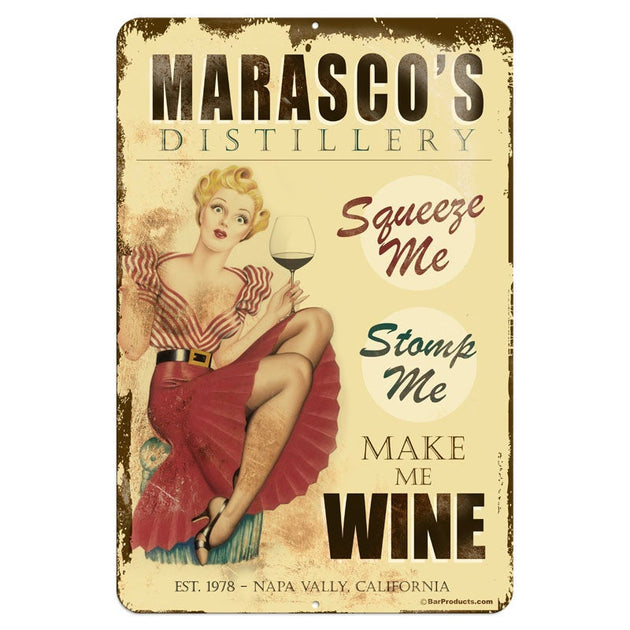The image is a vintage-style painted poster with a yellow background and brown edges, promoting Marasco's Distillery, established in 1978 in Napa Valley, California. Central to the poster is a woman with blonde hair and red lips, wearing a red and white striped top paired with a solid red skirt and a black belt with a golden buckle. She is seated, holding a glass of dark red wine and looking into the camera with a surprised expression. The text on the poster reads "Squeeze me, stomp me, make me whine" in various colors: "squeeze me" in red, "stomp me" in green, and other text in brown. Above the woman, the words "Marasco's Distillery" are prominently displayed, with "Marasco's" in dark brown and "Distillery" in a smaller green font. At the bottom, it states "Established 1978, Napa Valley, California," emphasizing the distillery's long-standing heritage.